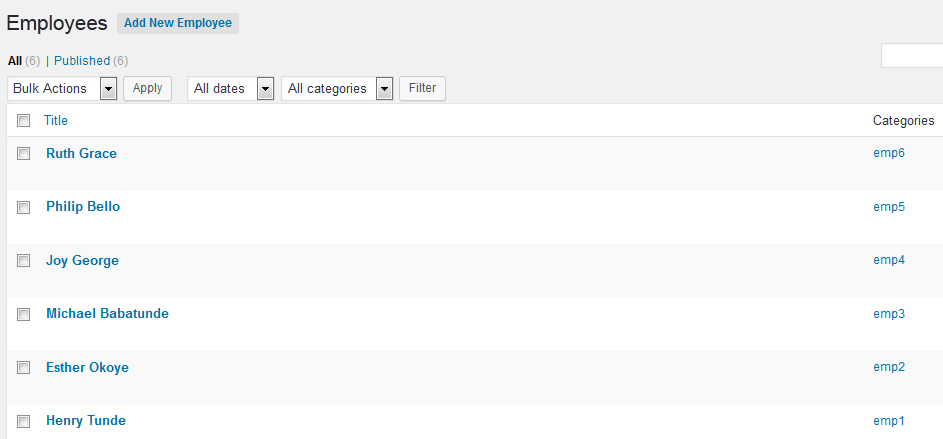The image depicts a website interface for managing employees. In the top left corner, the word "Employees" appears prominently in black. Just beside it, in blue text, is a clickable option labeled "Add New Employee." Below this, there is a note indicating a total of six employees, all published.

On the left side of the interface, there are several functional elements for bulk management: a drop-down menu labeled "Bulk Actions" followed by an "Apply" button. Additional drop-down menus labeled "All Dates" and "All Categories" are available to filter the employee listings, with a "Filter" button situated directly underneath.

The main content area displays a list of employee names, each styled as a blue link and alternating in gray and white background colors. The names listed are:
1. Ruth Grace
2. Philip Bellow
3. Joy George
4. Michael Badattu Undi
5. Esther Akoy
6. Henry Tundi

On the right side of each name, there is a corresponding "Categories" column, listing each employee with the label "Employee" followed by their respective numbers in descending order from six to one.

The overall appearance of the website is described as having a washed-out, subdued color palette, making it predominantly black and white with very light hues.